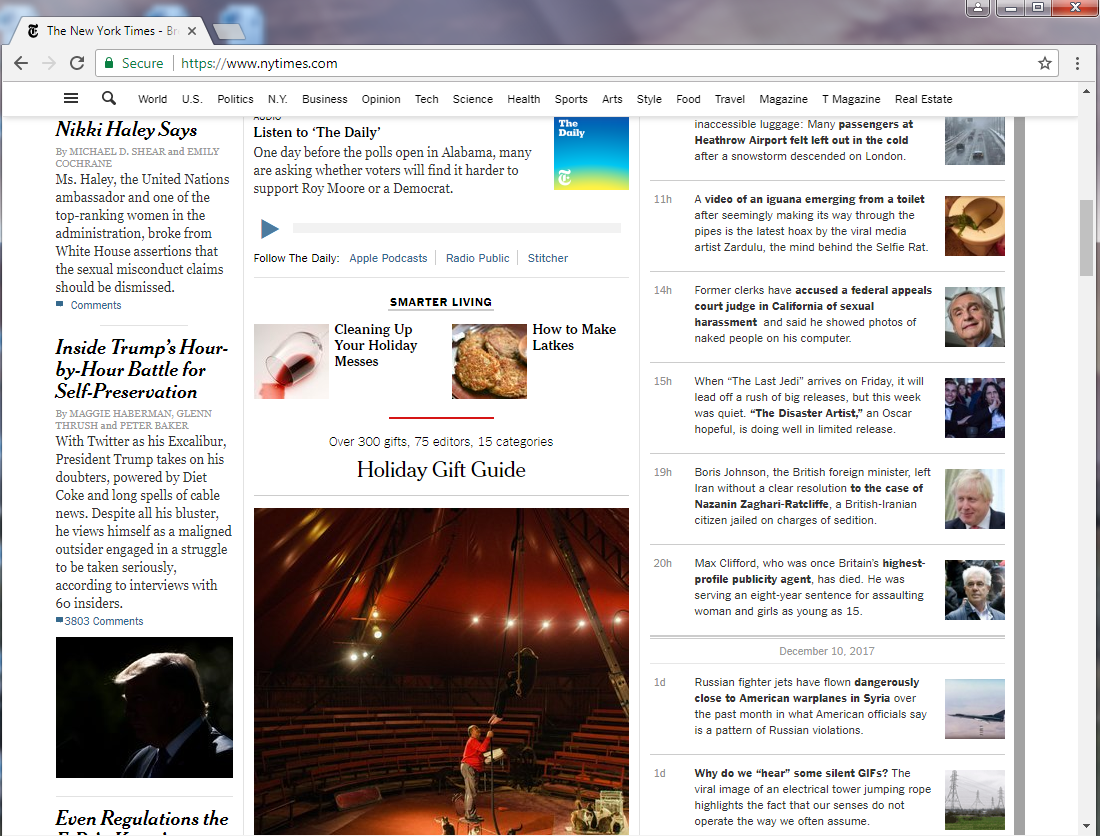This screenshot captures a webpage from the New York Times as viewed on an internet browser, potentially Safari. The browser interface is visible, featuring the New York Times in black text with a green 'secure' icon and HTTPS within the URL bar, which is white. The main content includes various articles, prominently displaying the headline "Nikki Haley Says" by Michael D. Shear and Emily Crane. Another leading story beneath this features "Inside Trump's Hour-by-Hour Battle for Self-Preservation."

On the right side of the page, there's a list of articles, accompanied by their respective posting times, which include timestamps such as 11 hours ago, 14 hours, 15 hours, and 19 hours. The far-right edge of the screen features a gray vertical scrollbar.

Towards the bottom center of the screenshot is an image of a person, framed within a circular area. The individual is looking upwards from red-themed surroundings that include red seats and a similarly hued ceiling adorned with small lights. The person is dressed in a red shirt and pants, seemingly reaching up towards something that’s not entirely clear. Additionally, there appears to be a cat or dog towards the bottom left of this image.

Adjacent to this image, positioned to the left under the headline "Inside Trump's Hour-by-Hour Battle," there's another photograph. This image showcases a partial view of Donald Trump with sunlight illuminating his hair, while the rest of the picture is largely shadowed.